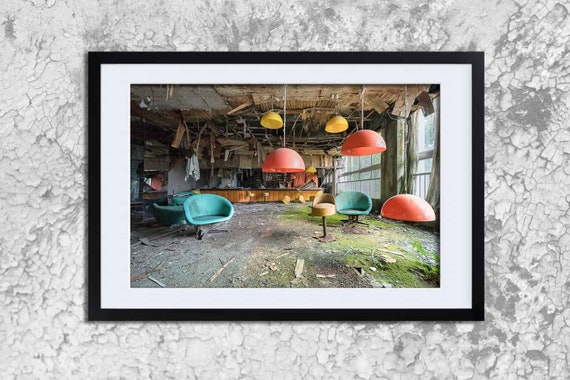This is a detailed photograph of a black rectangular photo frame hanging on a crumbling white and greyish wall. The wall itself has noticeable grey cracks and an irregular marble-like pattern. Within the frame is an image of a severely dilapidated room, where the walls and ceiling are falling apart and covered in various shades of white, grey, and tan. The room’s roof is partially caved in, and there is moss spreading across the uneven floor, which transitions from dirty brown on the left to different shades of green towards the right. Despite the disrepair, the room contains strikingly new, brightly colored modern furniture: two vibrant blue chairs with metal legs, a single yellow bar stool, and a mix of three red lamps alongside two yellow lamps hanging from the ceiling. Additionally, there's a cluttered background featuring what appears to be old books or manuals, and a brown bar can be seen in the background, further highlighting the contrast between the decayed setting and the pristine furniture.